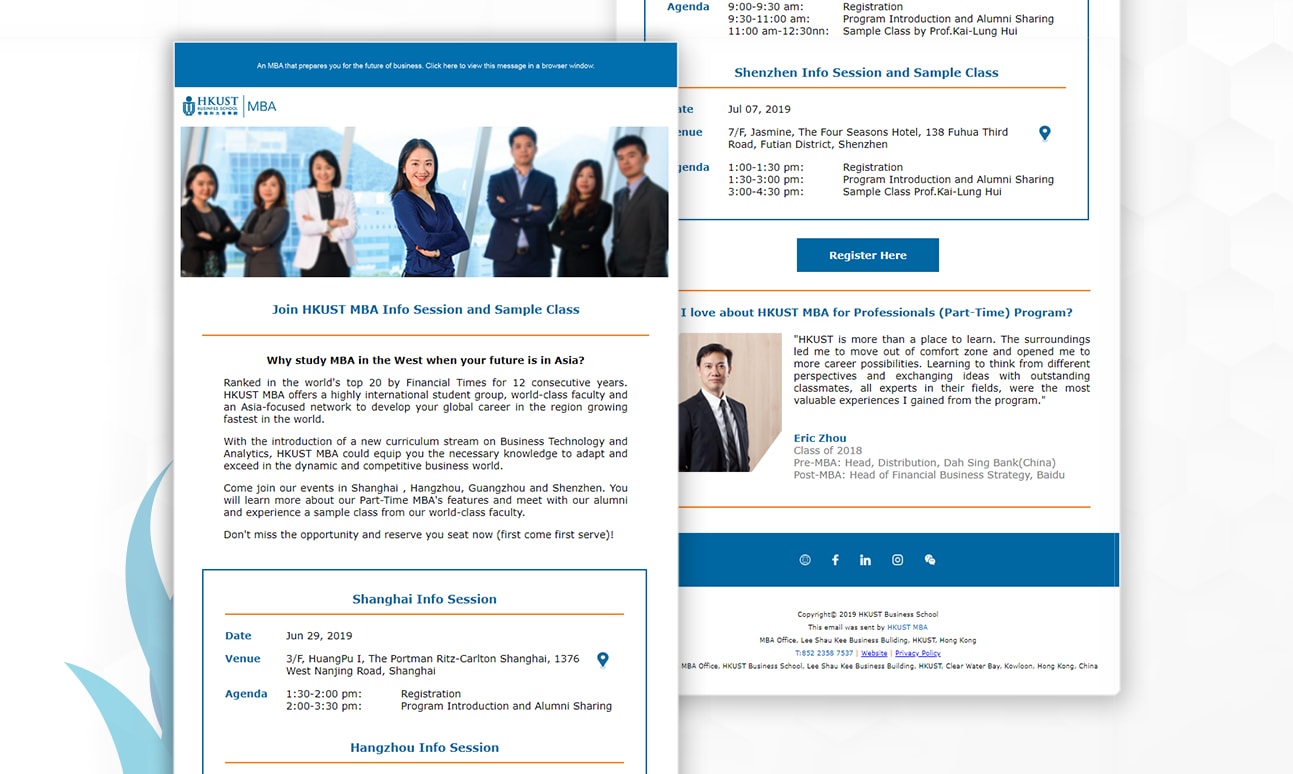The image is a promotional material for the HKUST MBA info session and sample class, featuring key event details set against a plain white background. A small section of teal-colored grass-like artwork appears on the left edge, adding a touch of color. The main content consists of two digitally generated pages displaying information about the event.

The HKUST MBA title is prominently displayed, accompanied by a photograph depicting a group of seven individuals, predominantly of Asian descent, standing in a well-lit room with large windows that offer a high-level view of the surrounding area. The group includes four women on the left side, and two men separated by another woman on the right side. The event specifically highlights the Shanghai info session held in China on June 29th, 2019, at the Portman Ritz-Carlton Shanghai. Key timings include a registration period from 1:30 to 2:00 p.m., followed by a program introduction and alumni sharing session from 2:00 to 3:30 p.m.

Additionally, the image lists similar events in Hangzhou and Shenzhen, along with their respective registration and program schedules. A testimonial from a CEO endorses the program, emphasizing the aspects he appreciates, which are highlighted as a part of the promotional effort.